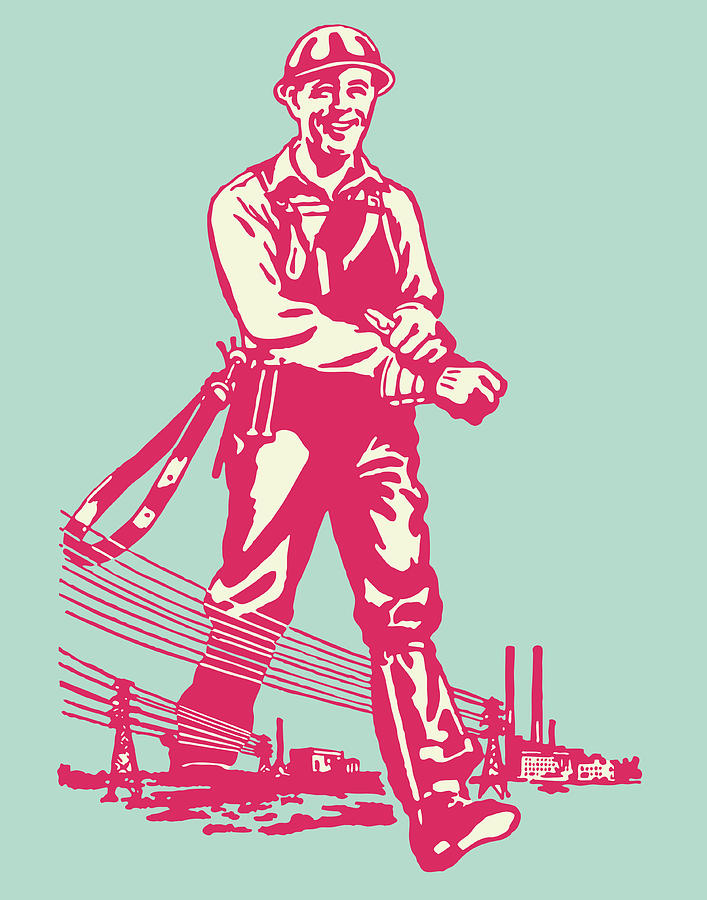This vertical rectangular drawing, rendered predominantly in shades of pink against a pale lime green background, depicts a towering man in worker attire. He wears overalls, a long-sleeved shirt, a hard hat, work gloves, and heavy shoes. His outfit includes a belt adorned with a loop, likely used for climbing telephone poles, emphasizing his role as a laborer. The man's confident smile and the dominating posture, with one foot in front of the other, conveys his mighty presence and power.

Running along the bottom of the image are power lines, which weave through his legs as he seemingly steps over them, further illustrating his colossal stature. The power lines stretch toward the left, originating from an industrial factory on the right, distinguished by its tall smokestacks. These elements underscore his significant role in creating and sustaining the depicted industrial landscape. The simplistic yet bold use of color and form—pink, cream, and minty green—adds a unique artistic touch to the powerful imagery.